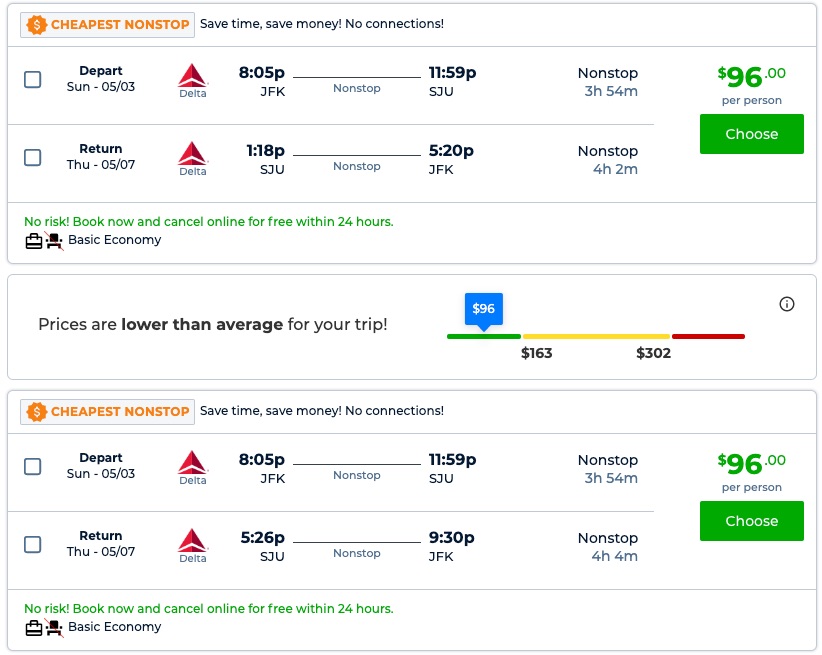A list of flights is displayed, highlighting the cheapest non-stop options to save time and money with no connections. The flight details are as follows:

- **Departure:**
  - **Day:** Sunday, May 3rd
  - **Airline:** Delta
  - **Time:** 8:05 PM
  - **From:** JFK Airport
  - **To:** SJU (San Juan) 
  - **Duration:** 3 hours and 54 minutes
  
- **Return:**
  - **Day:** Thursday, May 7th
  - **Airline:** Delta
  - **Time:** 1:18 PM (Departing SJU) 
  - **To:** JFK Airport 
  - **Duration:** 4 hours and 2 minutes

- **Pricing:**
  - **Cost:** $96 per person
  - **Book Now:** A green button for booking is provided, stating "No risk, book now. Cancel online for free within 24 hours" in green text.
  - **Fare Type:** Basic Economy
  - **Price Note:** The prices are lower than average for this trip, with $96 highlighted in green, and other prices listed as $163 and $302, with varying indications for price competitiveness (green for low, yellow for moderate, red for high).

- **Additional Information:**
  - **Highlights:** Emphasized messages include "Cheapest non-stop", "Save time, save money", and "No connections".

This organized format provides an efficient overview of the most cost-effective and time-saving flights available, making it easier to book a convenient travel option.